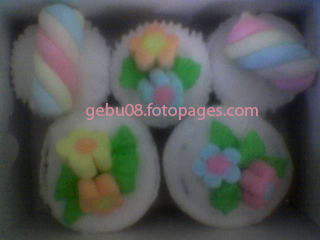The image is a small, slightly out-of-focus photo of five cupcakes arranged with three on top and two below, taken from a top-down perspective. Each cupcake is adorned with white frosting. The three cupcakes on the bottom showcase intricate pastel-colored flower designs, with each flower accompanied by leaves. The flowers are blue, pink, yellow, and orange. The two cupcakes on the top feature twisty, barber pole-like decorations in pastel shades of blue, pink, and white. Across the center of the image, in peach lettering, is the web address gebu08.fotopages.com. The overall quality of the picture is grainy and the details are somewhat obscured by the low light and blur.